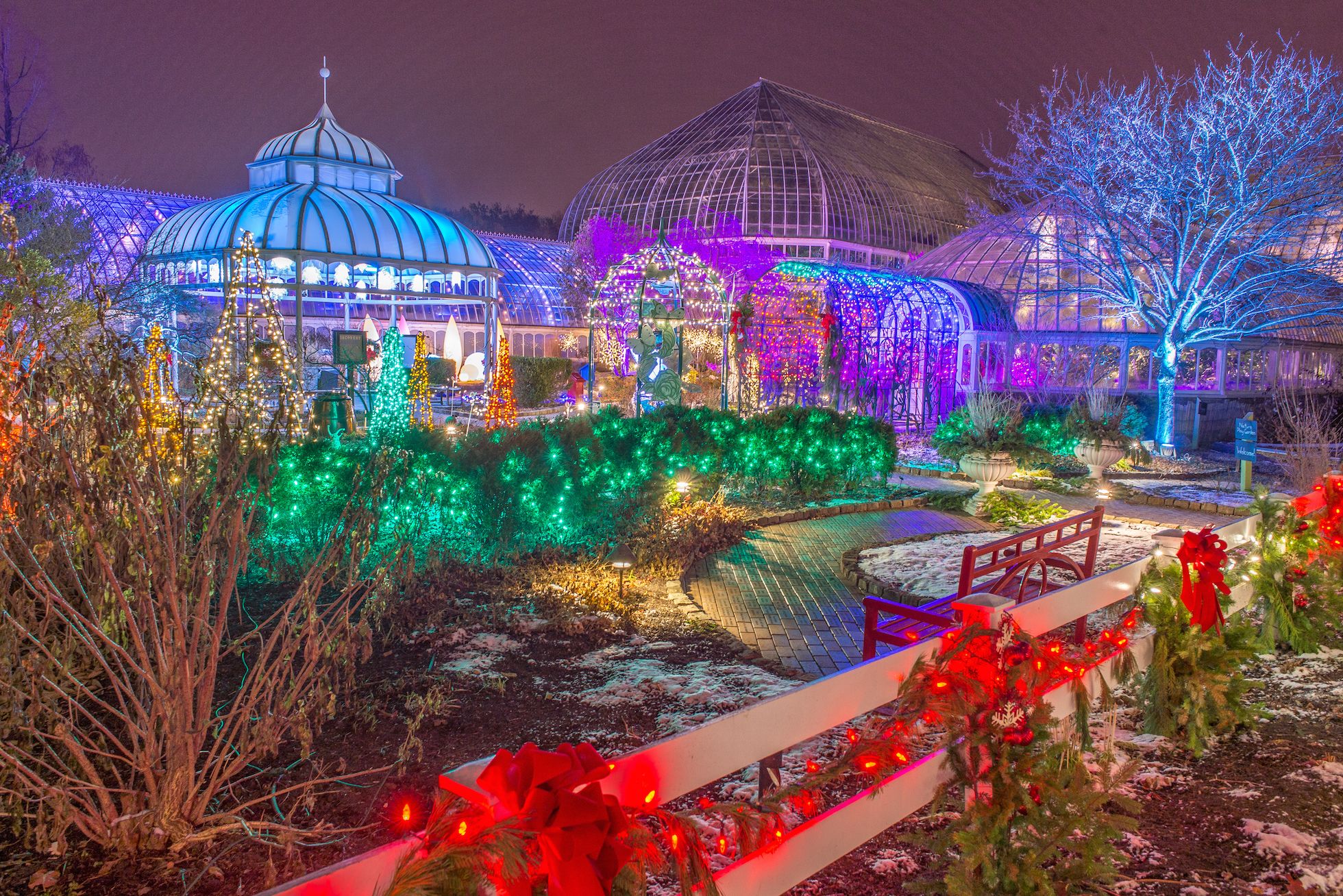This enchanting nighttime photograph captures a vibrant garden scene adorned with dazzling holiday lights. In the foreground, a white, wooden rail fence stretches diagonally from the middle right to the lower left, festooned with garlands of greenery adorned with red Christmas lights and elegant red bows at each post. Just in front of the fence, a paved area hosts a red park bench, inviting visitors to pause and take in the festive display. Flanking the bench is a hedge illuminated with bright green lights, adding to the holiday ambiance.

On the right side of the frame, a tree bathes in a soft blue hue, its glow evoking a wintry feel. Tall conical trees, one glowing green and the other white, rise behind the hedge. The center of the image features additional trees lit in purple and white, while an archway to the side is vividly illuminated in green, purple, and orange lights, creating a magical entrance.

In the background, three large glass structures resembling plant conservatories stand tall. These greenhouse-like buildings are constructed with glass panes supported by metal frameworks and emit a brilliant array of colors—purple, light blue, and white—casting an ethereal light over the scene. The dark sky above, tinged with a deep purple, provides a striking contrast to the myriad colors below, enhancing the festive, almost surreal atmosphere. Snow lightly dusts the ground, adding a final touch of holiday charm to this captivating tableau.